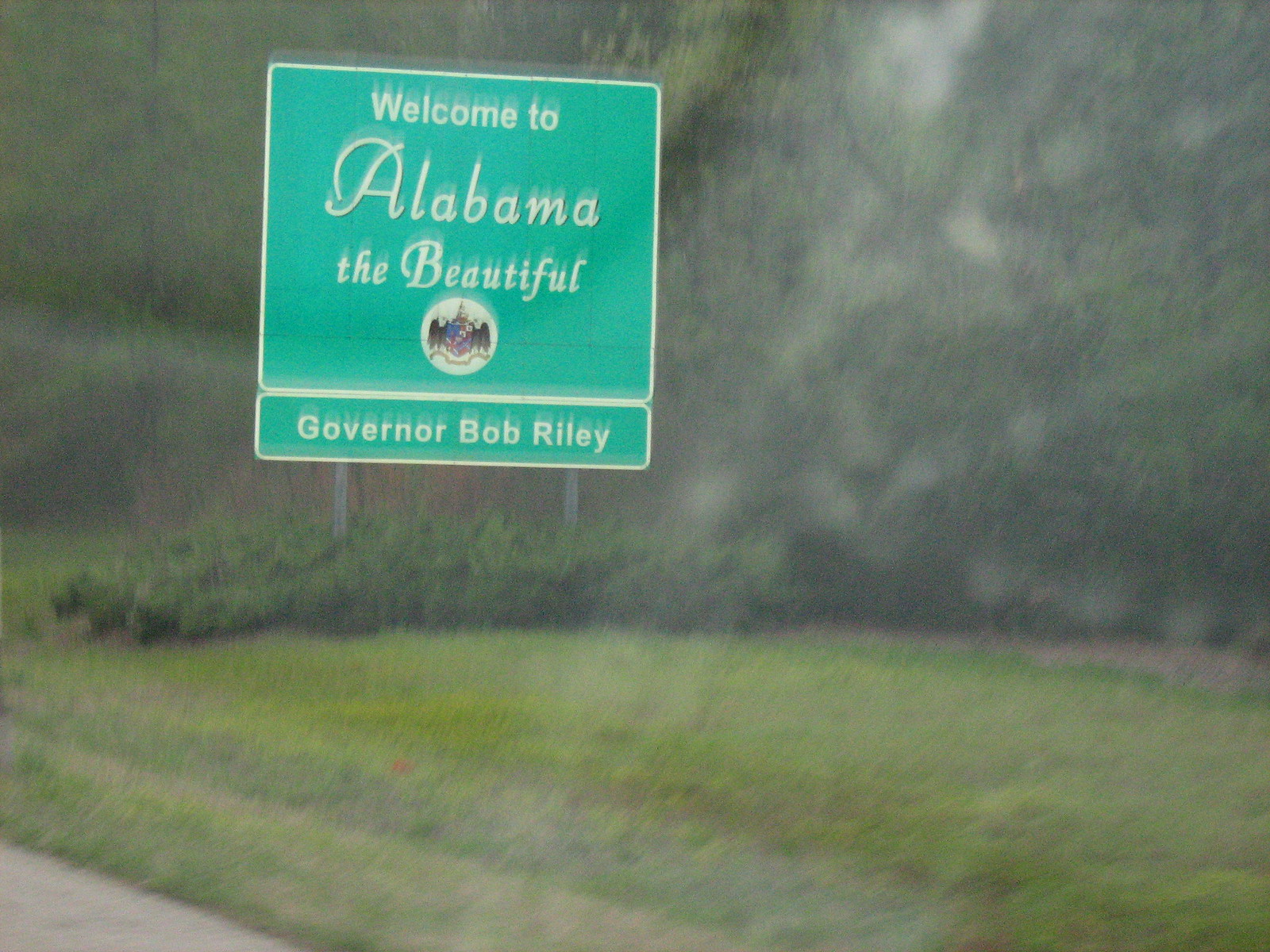The photograph captures a "Welcome to Alabama the Beautiful" street sign, prominently displayed against a backdrop of lush vegetation, including various trees and shrubs. The sign itself is green with white borders and features text in white, with "Alabama the Beautiful" written in an elegant script and the rest in a sans-serif font. At the bottom, it credits Governor Bob Riley. 

Additionally, the sign sports what seems to be the Alabama state logo, depicting a bird with a flag motif. The image, seemingly taken on a cloudy or rainy day, is shot through a car windshield, as evidenced by the faint reflections on the glass and slight blurriness hinting at inclement weather. The street sign is supported by two sturdy metal poles, securely placed in the ground.